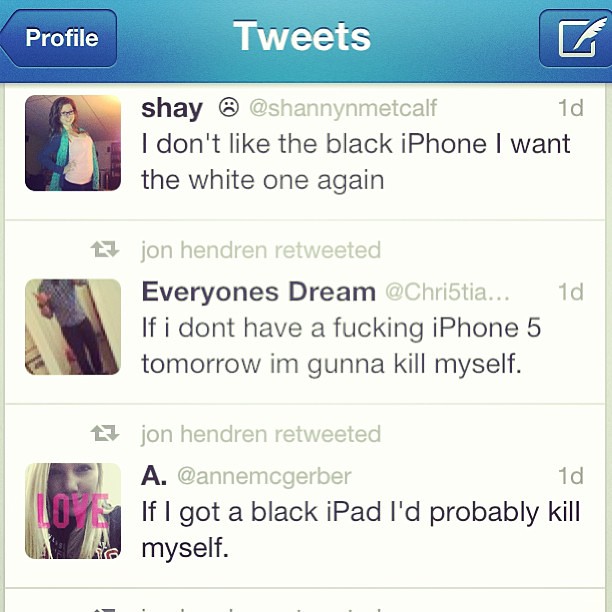This is a large square screenshot taken from a mobile phone, capturing an early version of Twitter, evident from the antique-looking fonts. At the top of the image, there is a blue bar with the word "Tweets" prominently displayed in white text at the center. To the left of this text is a "Profile" button, and to the right is an icon resembling a feather, likely meant for composing new tweets.

Below the blue bar with "Tweets," the image features three separate tweets, each with a small profile picture to the left. The leftmost tweet is from a user named Shay, whose name appears in bold black letters. Shay's tweet reads: "I don't like the black iPhone I want the white one again," and in the upper right corner, it indicates the tweet was posted one day ago (1D).

The middle tweet is from John Hendren, identified by the mention "retweeted" under his name, though only his body is visible as he stands in a doorway. His tweet states: "If I don't have a fucking iPhone 5 tomorrow I'm gonna kill myself," and it also notes "1D" in the upper right corner, indicating it was posted one day ago.

The final tweet features a woman with long blonde hair, her face partially covered with the word "LOVE" written in all-caps pink letters. This tweet is accompanied by the information that John Hendren retweeted it, as indicated by "retweeted" and his handle, @MacGarver. The content of the tweet reads: "If I got a black iPad I'd probably kill myself," and it was likewise posted one day ago.